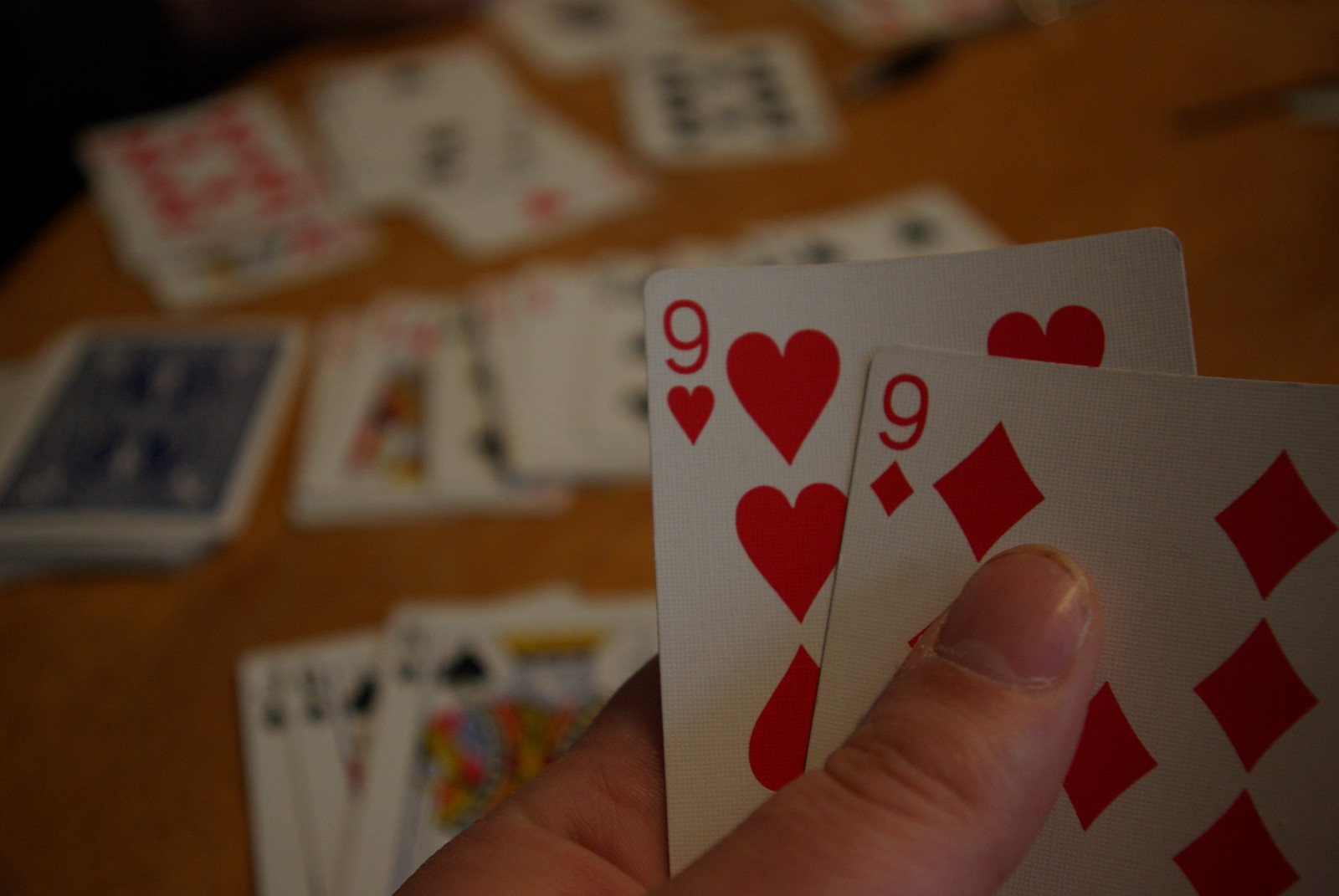In this high-quality photograph, a hand is prominently holding two playing cards – the nine of hearts and the nine of diamonds, both in vibrant red suits. The thumb, notably dirty, is resting on the nine of diamonds, adding a stark contrast to the otherwise clean and crisp imagery of the cards. The background features a blurred brown wooden table cluttered with additional cards, most of which are face-up, making it difficult to discern their exact details. To the left, there’s a larger pile of face-down cards. In the upper right corner of the image, there’s a blurry object that resembles a pen, further contributing to the scene's casual yet cluttered setting.